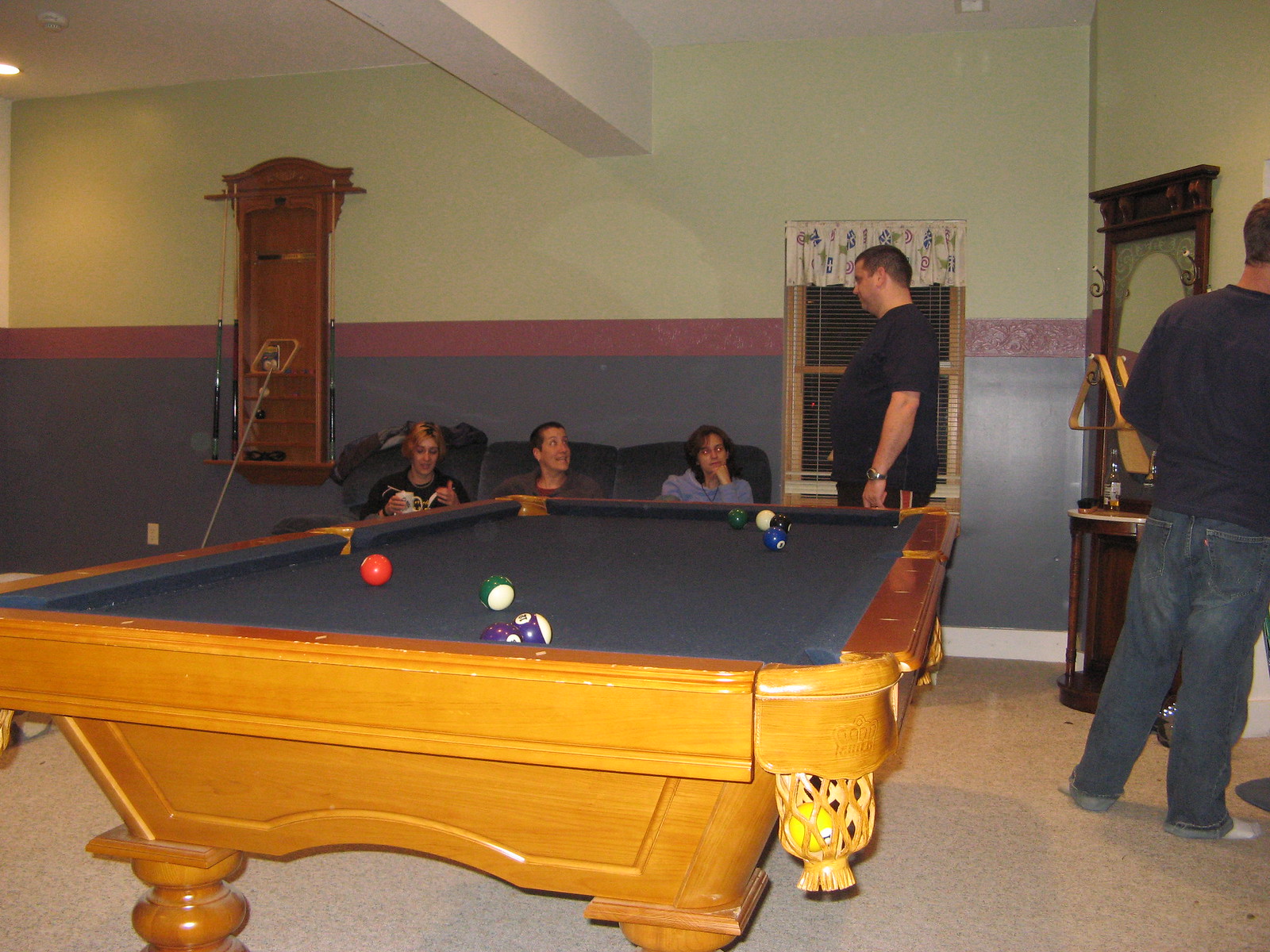This image captures a cozy entertainment room, possibly a basement converted into a man cave. Central to the room is a vintage pool table with beautifully carved, golden-brown wood and blue felt, lending a classic touch to the space. Several billiard balls are scattered on the table, and the pocket nearest the viewpoint holds a yellow pool ball.

In the far corner of the room, a woman and two men, likely in their 20s, are seated on a spacious, comfy couch. To their left stands a functional pool cue holder stocked with cues. An antique stand with a mirror and small tabletop, along with books, serves as a decorative yet practical piece, positioned flat against the wall.

Two men are positioned near the pool table, one in blue jeans and a sweatshirt standing near a window. He is casually conversing with the group on the couch, while another man in blue jeans and a blue shirt stands to the far right, engaged in a different conversation. The room also contains a unique exercise setup involving a wall-mounted piece that users sit on the ground to pull.

The overall atmosphere is warm and inviting, enhanced by brown carpeting and thoughtful placement of furniture and decor, making it an ideal space for relaxation and socialization.